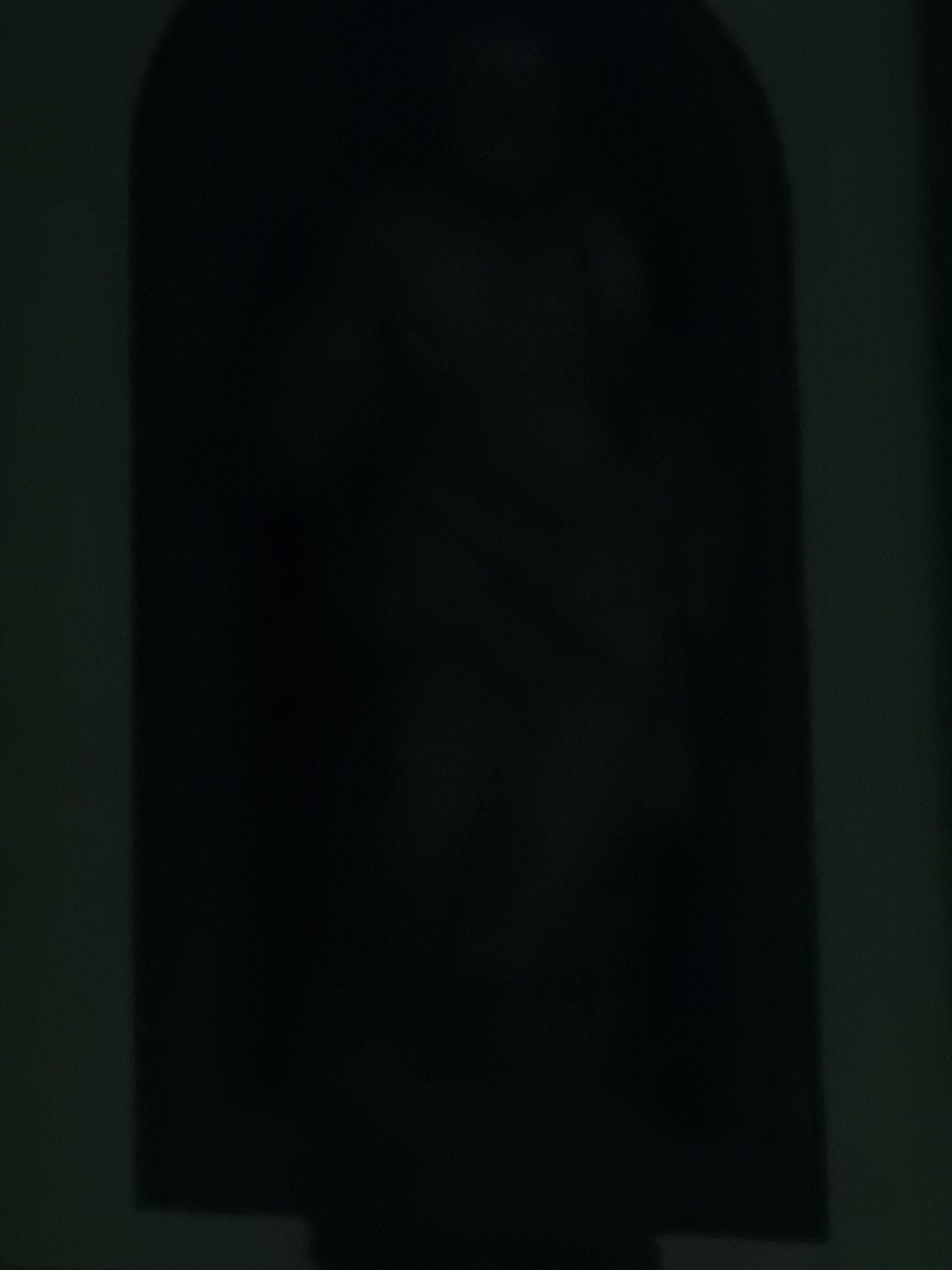The image features a predominantly solid black background, extending uniformly from top to bottom and left to right. Subtle variations in the black hue are present, particularly toward the corners and edges. In the lower right corner, there is a barely perceptible lightening, with the black transitioning to a very dark gray. This faint lightening effect extends along the bottom edge of the image and is similarly echoed in the lower left corner, which is slightly lighter than the central area. Additionally, the top edge and upper sides exhibit minimal lightening, creating a subtle gradient effect just at the periphery of the image. These nuances in shade are extremely faint, making the background appear almost entirely black at first glance.